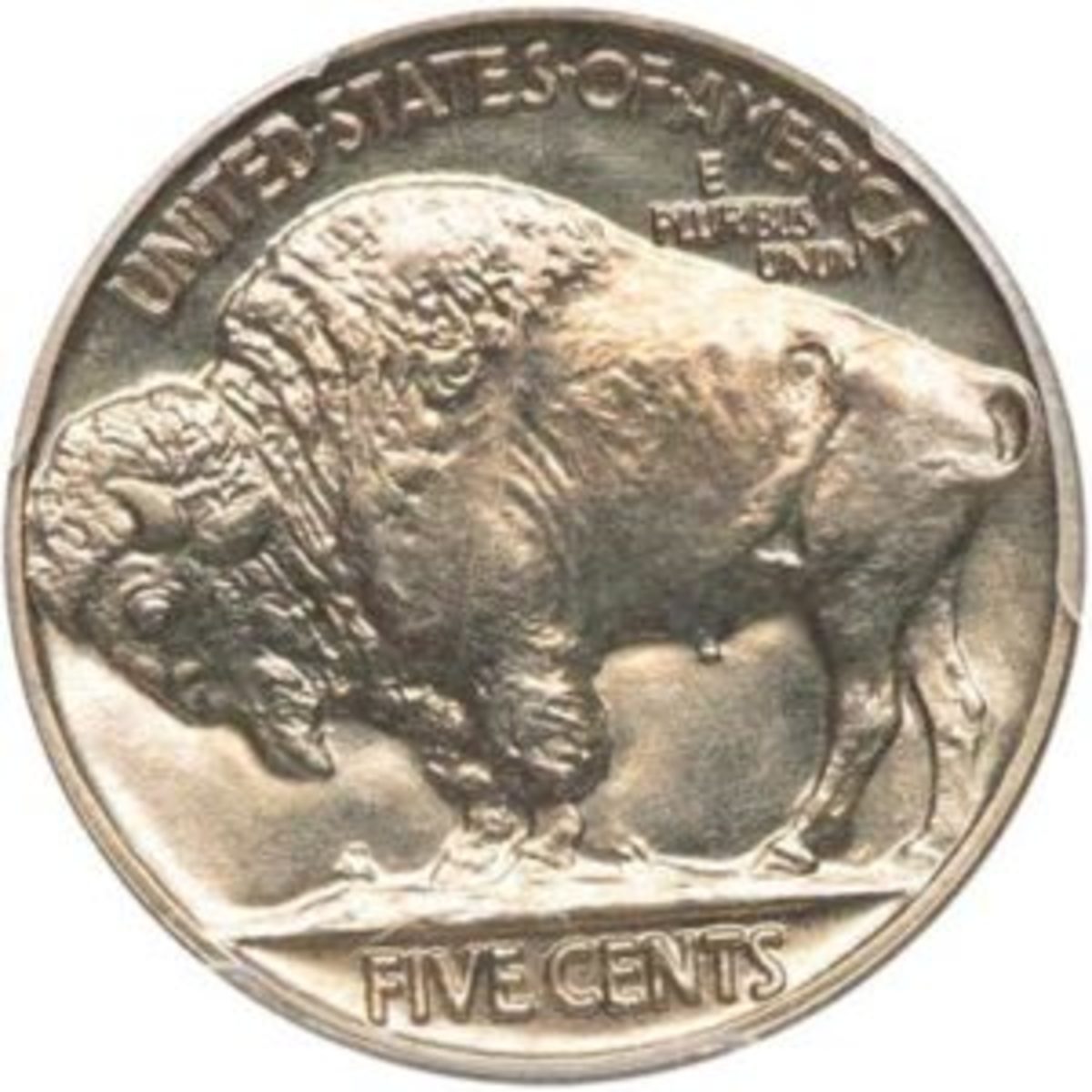The image showcases a close-up of a worn and slightly discolored coin, traditionally known as the buffalo nickel or bison 5-cent piece minted by the United States Mint. The coin, primarily silver with areas appearing brown due to age, features the inscription "United States of America" at the top, followed by "E Pluribus Unum," the official motto of the United States. Dominating the center is a detailed side profile of a male buffalo, identifiable by anatomical features, with its head lowered, horns visible, and tail curled. The buffalo stands on a textured ground with the denomination "Five Cents" inscribed below. Surrounding the coin is a small, slightly chipped border, adding to its aged appearance. The photograph quality is somewhat low, with a white background highlighting the coin's weathered condition.